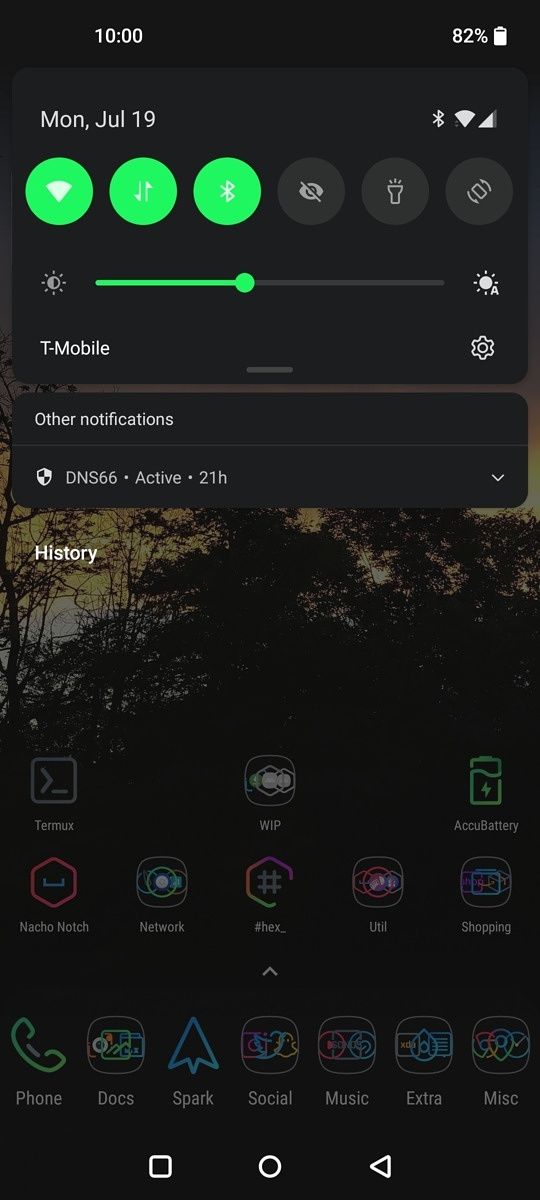This is a detailed color image of a cell phone screenshot, displayed in a rectangular format with a vertical orientation. At the very top of the screen, the status bar indicates it's 10:00 AM, and the battery charge is at 82%. Directly beneath this, the date is displayed as Monday, July 19th. To the right, icons show that Bluetooth is enabled, signal strength is present, and Wi-Fi is turned on.

Below this status bar, there are six circular icons aligned in a row. At the left end, three icons are filled with a solid green color, indicating they are active: Wi-Fi, download image, and Bluetooth features. The remaining three icons on the right are gray, signifying they are inactive: the flashlight is off, screen rotation is off, and possibly the camera is off.

Further down, the screen brightness slider is positioned slightly to the left of the center, allowing moderate screen brightness. Below this slider, "T-Mobile" is clearly written in white text, followed by a section labeled "Other notifications."

Within this section, there is a notification for an app named "DNS 66," which has been active for the last 21 hours. Just beneath this, there is a heading labeled "History."

The background of the screenshot features a very dark image which appears to be of a tree, adding a subtle yet visually appealing touch to the overall layout.